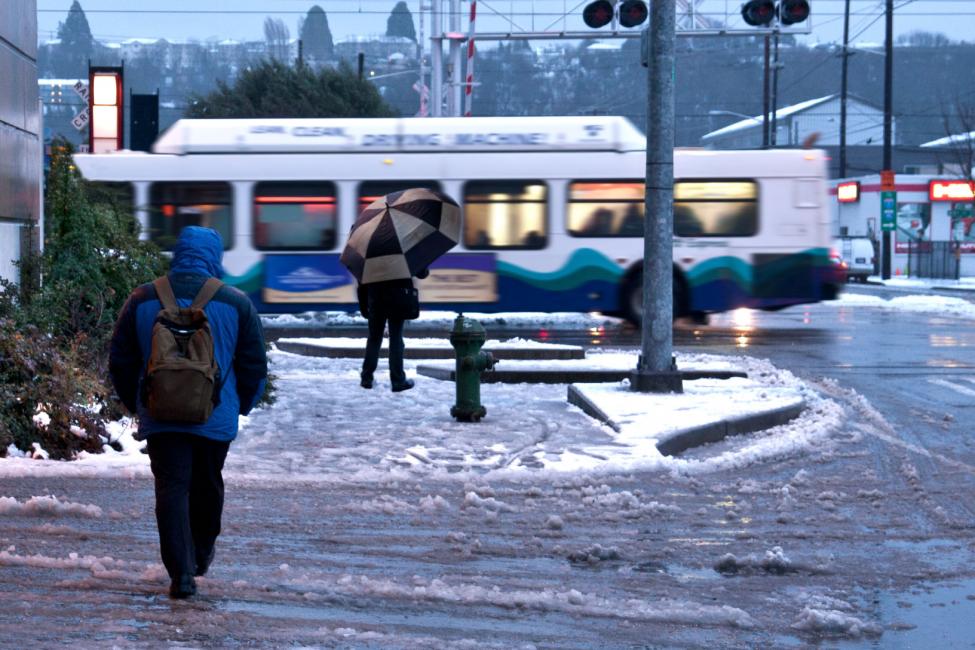In this detailed city scene on a cold, slushy winter day, two people are captured walking down a wet and icy street. The melting snow has turned the sidewalks and roads into a slushy mess. The person walking away from the camera is wearing a blue and green coat, carrying a brown backpack. Beside them, another individual, dressed in a black coat and slacks, is holding a tan and black umbrella. In the background, a white city bus with a wavy blue and green design along its lower half is passing by. The partially blurred signs on the bus read “clean drying machine.” To the right, there's a convenience store with an orange and white sign, and a green fire hydrant is positioned on the edge of the sidewalk. A railroad crossing complete with tracks and signal lights is also visible, along with an evergreen bush offering a touch of green amidst the otherwise gray, snowy landscape. The distant background reveals rows of trees, a hint of mountain terrain, and various building rooftops, including one likely signifying a laundromat. Overall, the scene reflects a dreary, bustling winter day in the city.